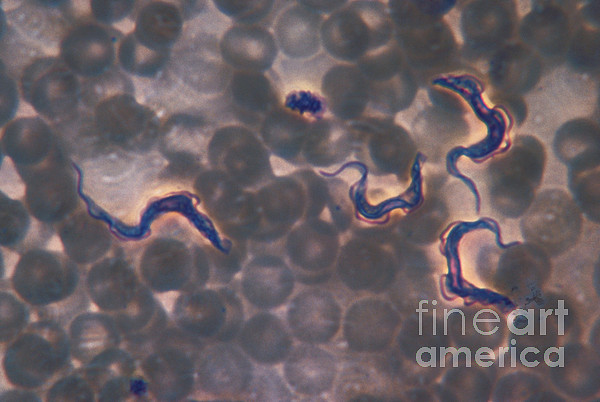The image appears to be a detailed, microscopic view featuring a variety of round and elongated objects. Dominantly grey and purplish in tone, the scene is reminiscent of a cluster of spherical bodies, possibly eggs, dispersed across the frame. Among these are several dark blue, worm-like formations—three closely grouped and one separated off to the side—as well as a small, bean-shaped object. These worm-like structures exhibit a slight pinkish hue along their edges. The background is predominantly dark, adding a sense of depth to the image. The text "Fine Art America" is discreetly placed in the lower right-hand corner. The overall aesthetic of the image is one of natural scientific beauty, suggesting an illuminated sample under a microscope.